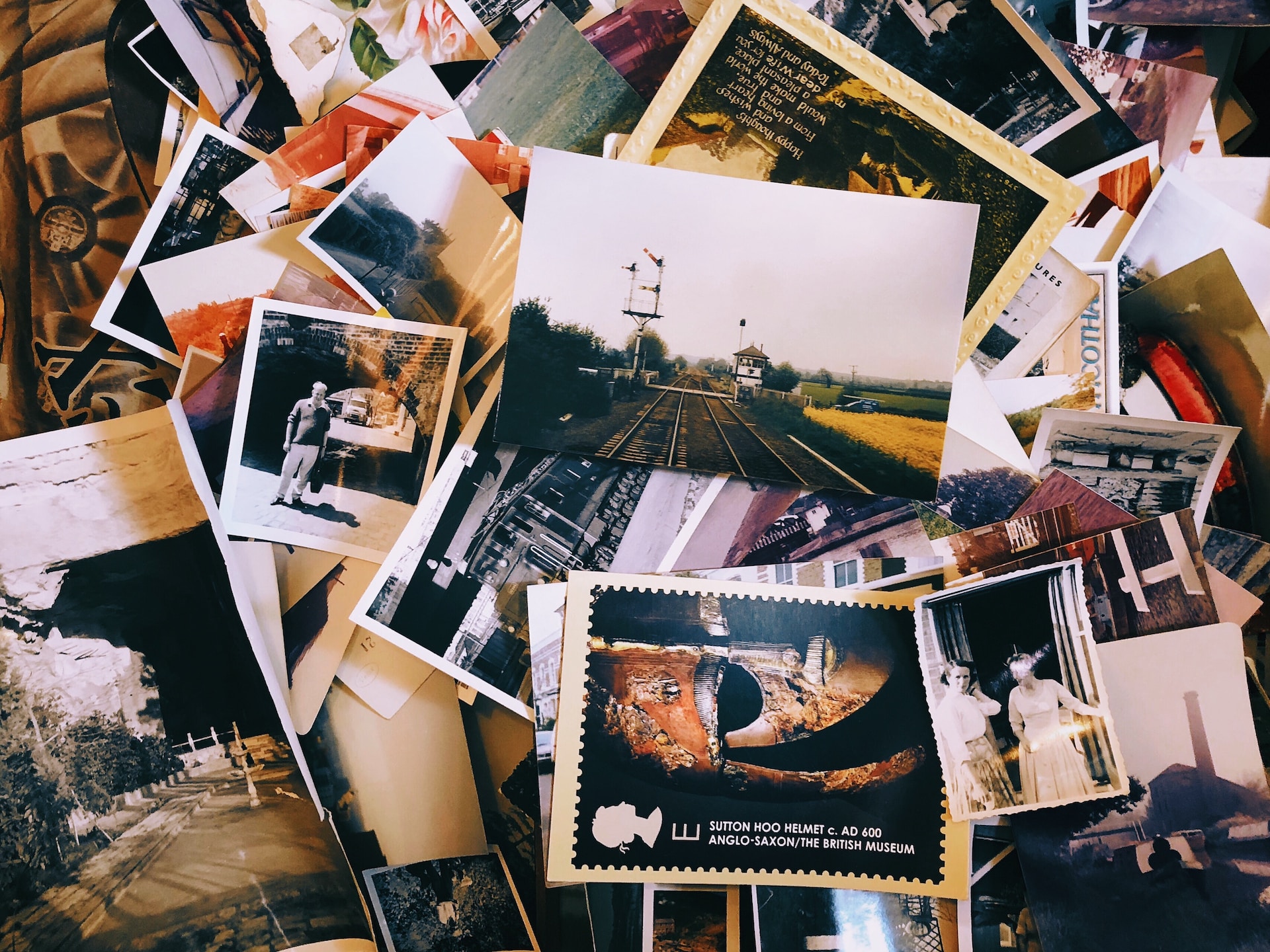The image depicts a chaotic assemblage of aged photographs, postcards, Polaroids, and magazine pages, all piled atop one another in a disorderly manner. At the upper-middle section, a prominent photograph featuring railroad tracks and a vast expanse of sky stands out clearly. Just to the left of this, an old, slightly cut-off black and white Polaroid shows an individual standing in front of a building. Below the railroad tracks image, there's a somewhat legible postcard displaying text that reads "Sutton Hoo Helmet, Anglo-Saxon, the British Museum," although the corresponding picture is indistinguishable. To the right, another black and white Polaroid depicts two women standing in a doorway. In the bottom left corner, a larger item, likely a magazine page, is visible, showing a scene with a sidewalk, built-up wall, and some trees. The collection features a mix of black and white and colored images, with many photos partially obscured, emphasizing the haphazard nature of the assortment.